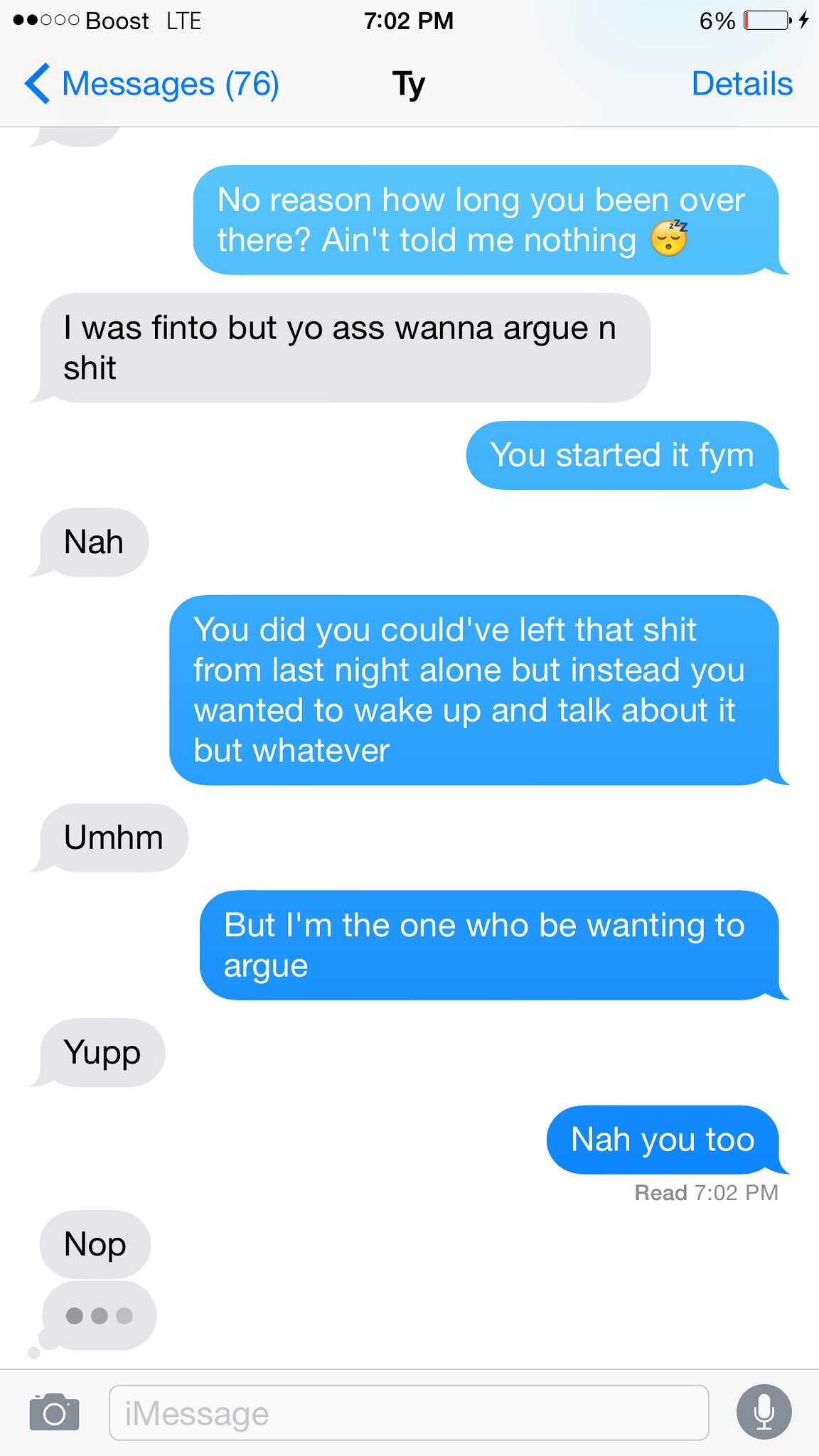The image depicts a text message conversation on a Boost LTE phone with 6% battery remaining, indicated by a drained battery icon with a red line and a lightning symbol. The screen shows it is 7:02 PM, and the messages count reads 76. The conversation starts with a blue bubble that reads, "no reason, how long you been over there, ain't told me nothing," accompanied by a sleeping emoji with blue Z's and a yellow face. The responses in gray and blue bubbles follow: "I was fit to, but yo ass wanna argue and shit," then "you started it, FYM," then "nah," then "you did, you could’ve left that shit from last night alone, but instead you wanted to wake up and talk about it, but whatever." This is followed by responses in alternating colors: "uh-huh," "but I'm the one who will be wanting to argue," "yep," "nah, you too," and "nope." Three dots in a gray bubble indicate an incoming message. At the bottom, the message box, a gray camera icon on the left, and a gray microphone icon on the right are visible, suggesting an ongoing text exchange between two individuals.